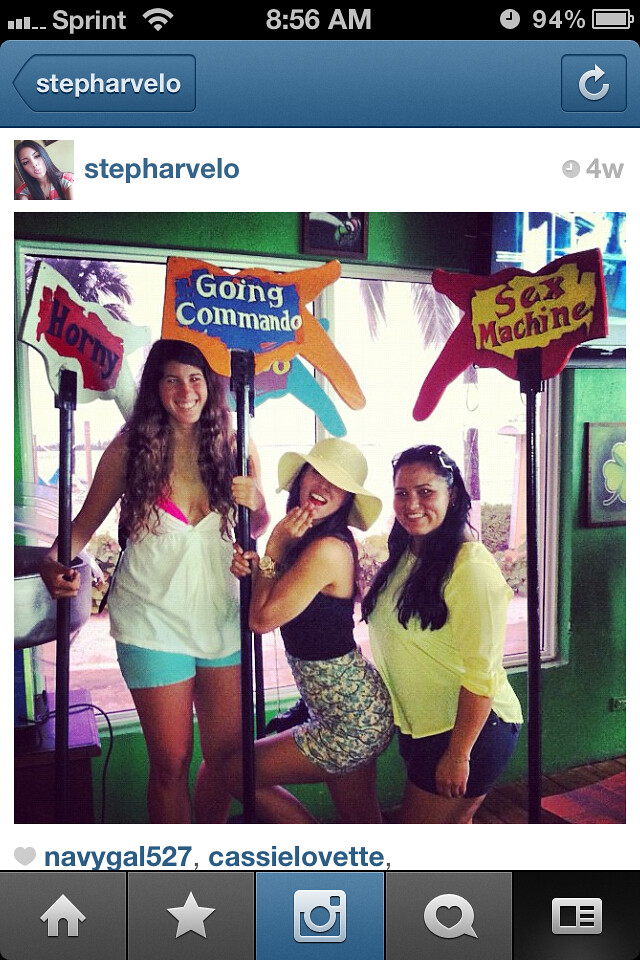The image is a screenshot taken from a Sprint phone displaying a social media post on Facebook at 8:56 a.m. with a battery level of 94%. The post is from an account named "Steph Avello." The picture shows three women standing in front of a dark green shop window, each holding a humorous sign. The woman on the left, who is tall with long dark brown hair, is wearing a white sleeveless top with a pink bikini underneath and blue shorts; her sign says "Honey." The woman in the middle, who has short black hair and a beige hat, is wearing a black sleeveless top and a tight multicolored skirt; her sign reads "Going Commando." The woman on the right has long black hair, a yellow short-sleeve shirt, and dark blue shorts; her sign says "Sex Machine." Each woman has distinct accessories, with the one in the middle notably wearing a golden watch on her wrist.